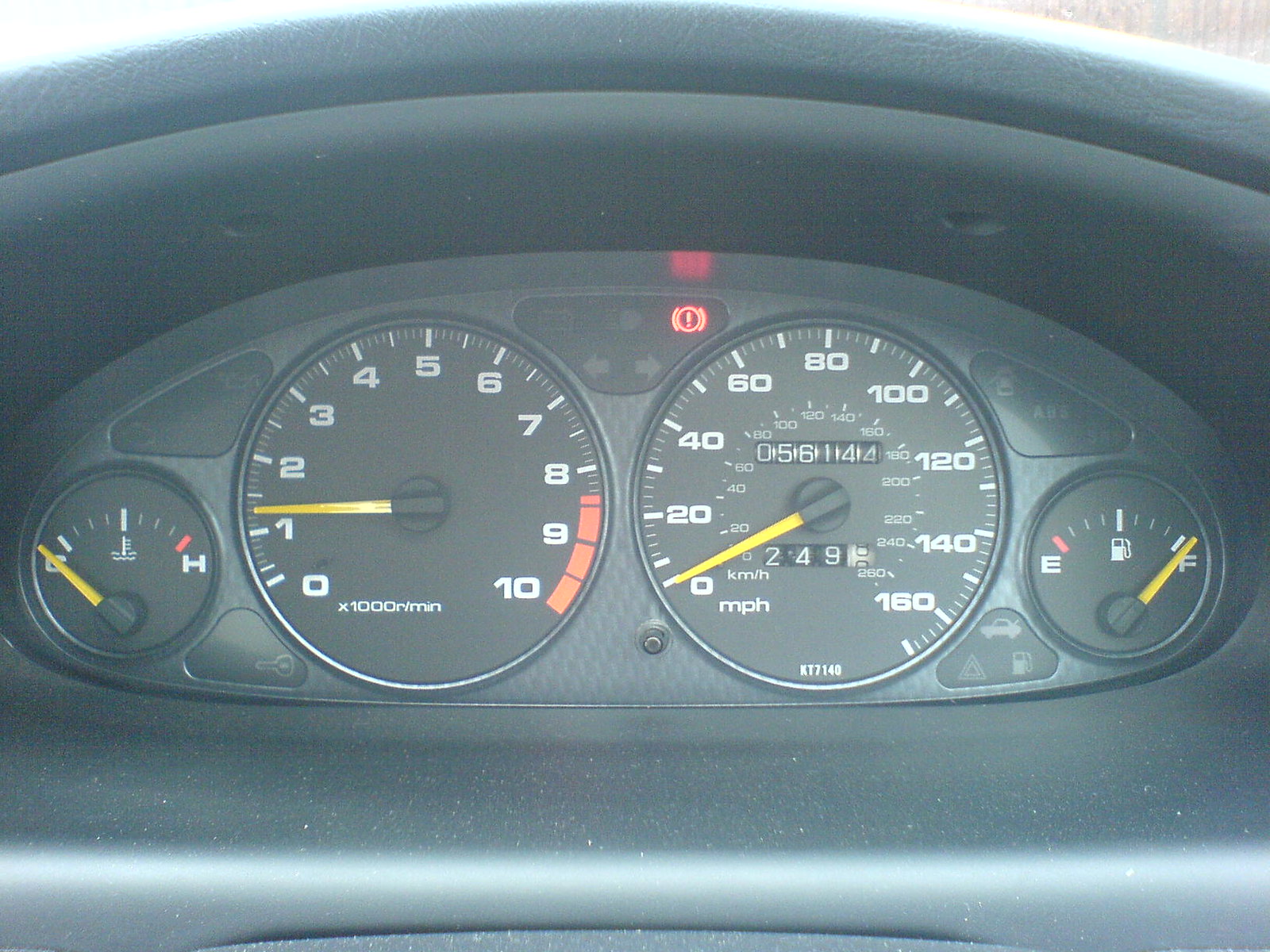This image showcases the dashboard of a vehicle, likely a motorcycle or a car. The dashboard features four distinct circular gauges. 

1. The first gauge on the left displays the temperature of the engine or another crucial vehicle component. It has markings indicating 'Cold' on the left and 'Hot' on the right, with a thermometer-like icon in the center.

2. The second gauge from the left is a tachometer, measuring the engine's revolutions per minute (RPM). It ranges from 0 to 10, with the text "×1000 RPM" inscribed on it.

3. The third gauge is the speedometer, which shows the vehicle's speed in miles per hour (MPH), ranging from 0 to 160. Within this gauge, there is a smaller, secondary scale for kilometers per hour (KPH), ranging from 0 to 260.

4. The final gauge on the right measures the fuel level in the vehicle's tank. This gauge indicates the fuel level from 'E' for empty to 'F' for full.